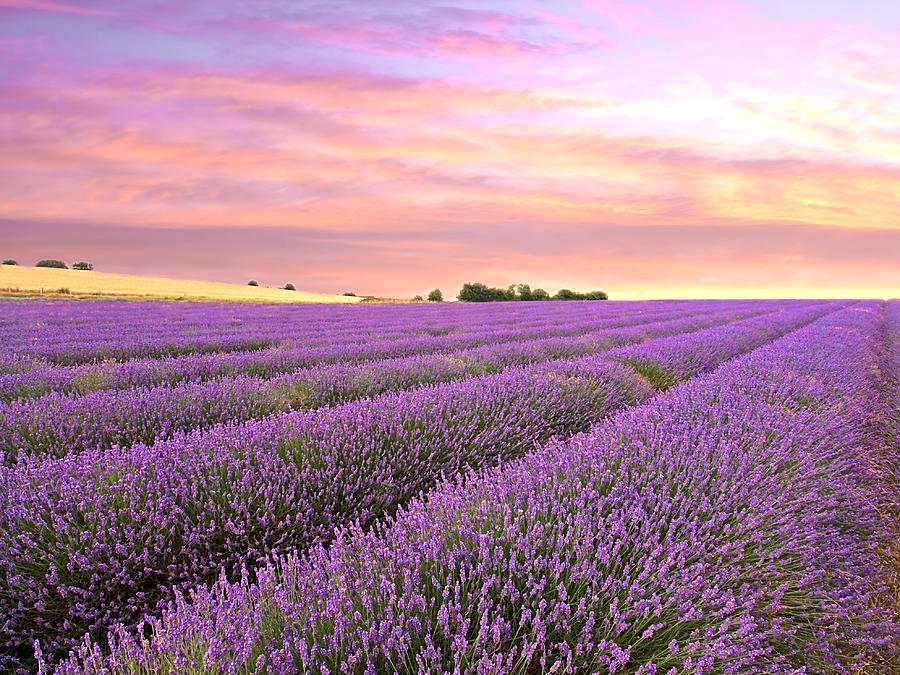This square, full-color photograph, captured outdoors during either sunrise or sunset, showcases a stunning and expansive field of purple wildflowers. The upper 40% of the image is dominated by a mesmerizing sky filled with a blend of colors - vibrant red, purple, pink, and orange clouds with golden-yellow hues, alongside patches of bright white and subtle blue. The sky is an exquisite backdrop highlighting the setting or rising sun's glow.

Below this dramatic sky, the scene transitions into an intricate landscape of over a dozen rows of small purple flowers with green stems and leaves. These flowers, identified by their narrow grass-like tips covered in blooms, are organized in neat rows with visible walking paths between them, extending towards the upper right corner of the photograph. To the left side of the frame, a tan patch of land can be seen, possibly another crop, contrasting against the vivid green and purple of the flowers. A line of distant trees frames the fields on the horizon, adding depth and context to this beautiful natural setting.